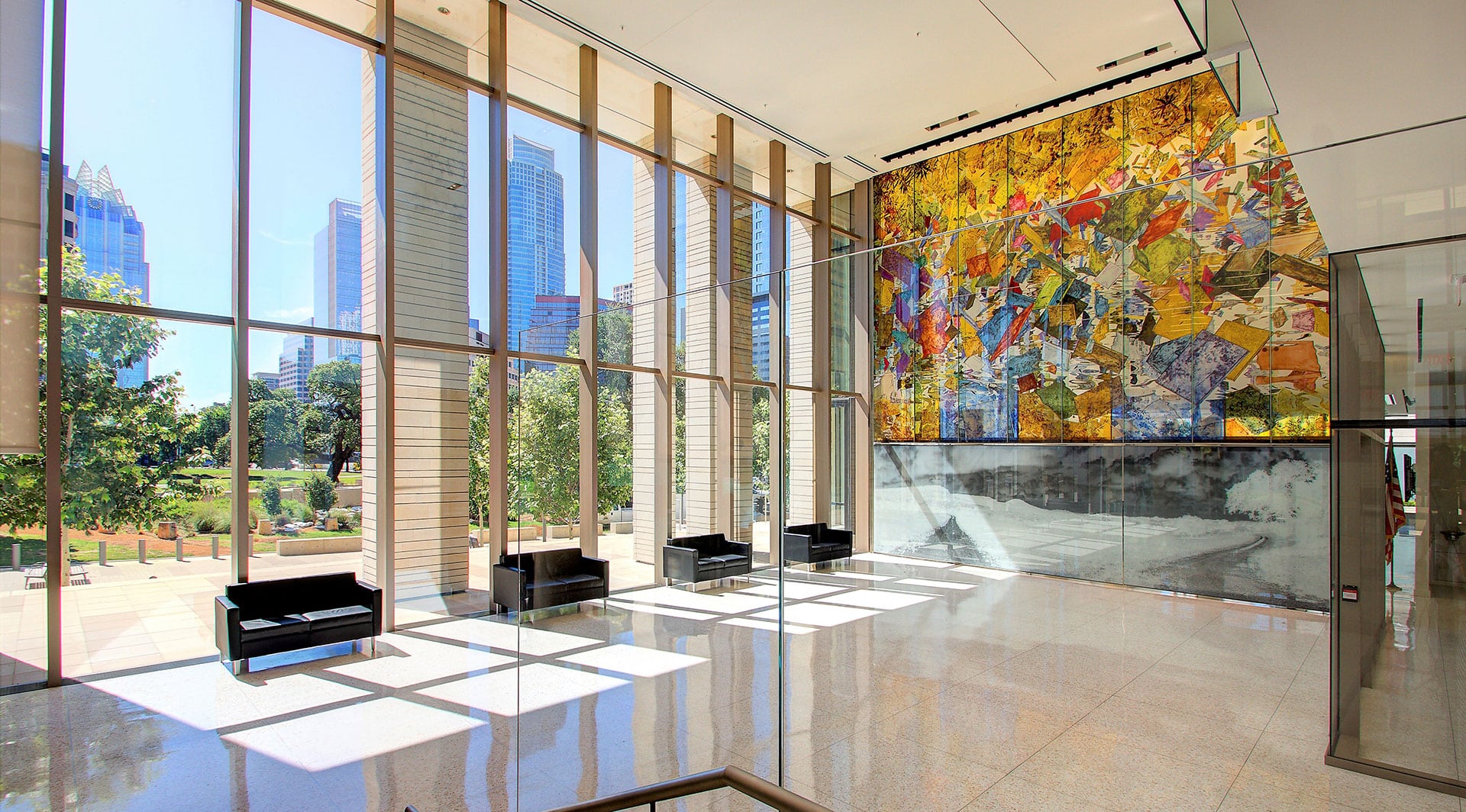This image captures a spacious, light-filled room within a predominantly glass-walled building, suggesting it might be an office space or lobby area. The white-painted interior features expansive, floor-to-ceiling windows on the left side that offer a view of trees, green spaces, and distant buildings. The floor is covered with large, white tiles. In front of the windows are four black chairs arranged to face inward. On the right side of the image, a vibrant mural with colors such as green, red, blue, yellow, and purple adorns the wall, above a black-and-white piece of artwork at the bottom. To the far right, the American flag is visible through glass partitions leading into another room. The room's high ceiling, painted white, adds to the open and airy atmosphere.